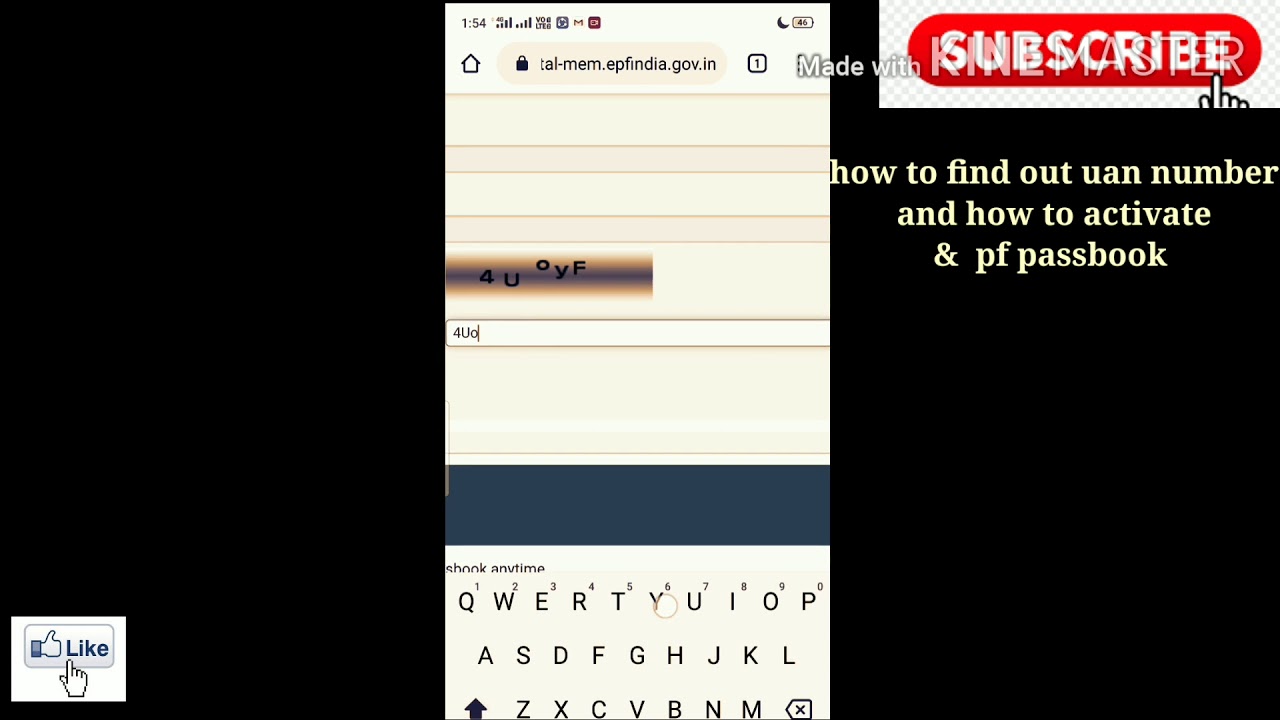The photograph displays a slightly disorganized web page. On the far right side, the word "subscribe" is prominently featured in red, accompanied by a small hand icon pointing towards it. Below this subscription prompt, there's a yellow text box in lowercase letters reading "how to find out UAN number and how to activate and PF passbook."

At the center of the image, there appears to be a screenshot likely taken from a smartphone. The top bar of the screenshot shows various indicators such as the current time, Wi-Fi signal strength, cellular signal strength, a moon icon (indicating Do Not Disturb mode), and a battery icon showing 46% charge. In the middle, a partial web address is visible: "T-A-L/M-E-M.E-P-F-I-N-D-I-A.gov.in," suggesting the website is related to India.

The page displayed on this screenshot features a CAPTCHA challenge with the code "4U0YF," which has been partially typed into the corresponding input field. Below the CAPTCHA input, there is a typical smartphone keyboard in QWERTY layout with some numerical keys and a prominent black arrow key.

To the far left of the photograph, a like icon is noticeable, with a small hand icon pointing towards it, indicating an option to "like" the content.

The web page's background is predominantly black, while the elements and details mentioned are set against this contrasting backdrop, creating a distinctive and cluttered visual presentation.